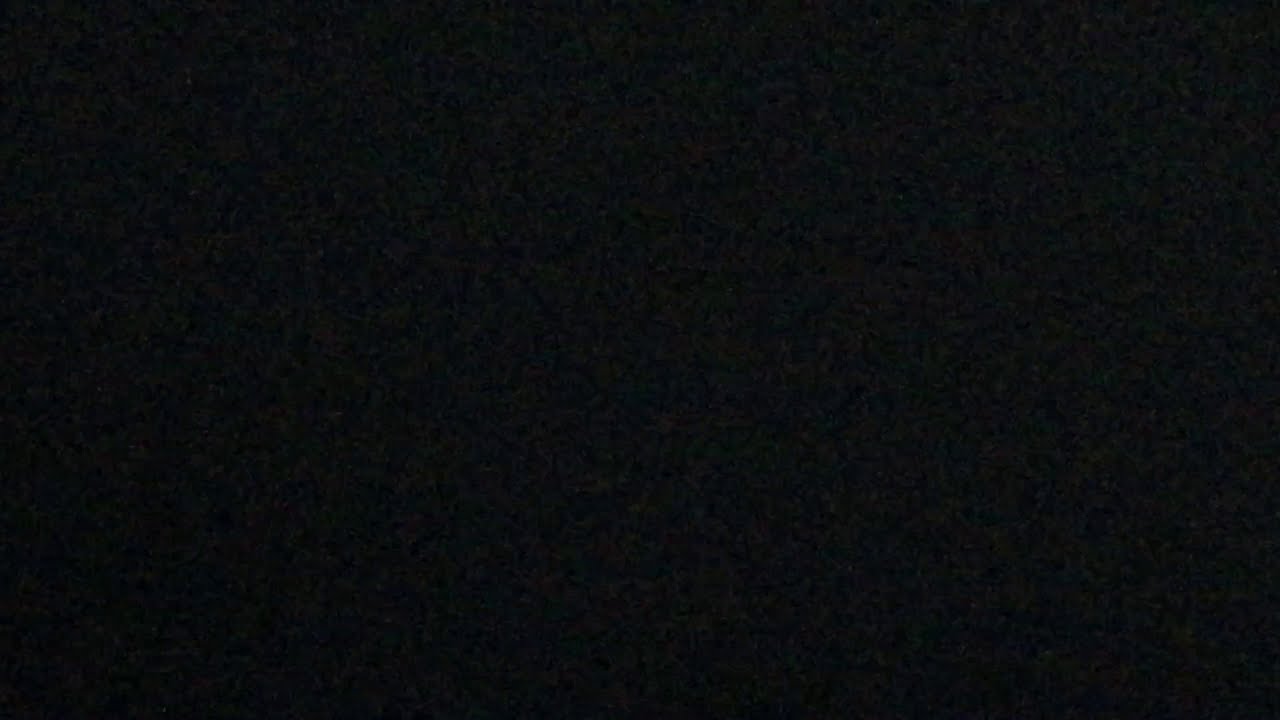The image depicts a predominantly black rectangle that brings to mind a TV screen displaying static, characterized by its textured appearance. While the rectangle appears almost solid black, closer inspection reveals an array of subtle, lighter hues, including shades of gray, white, and faintly noticeable reds, interspersed throughout, giving it a sense of random static. Despite these details, no discernible pattern or design can be clearly made out. The rectangle is bordered by a thin rim and surrounded by a small circular shape, adding to the sense of abstraction. Overall, the image evokes a sense of ambiguity and resembles a screen caught in a moment of static.